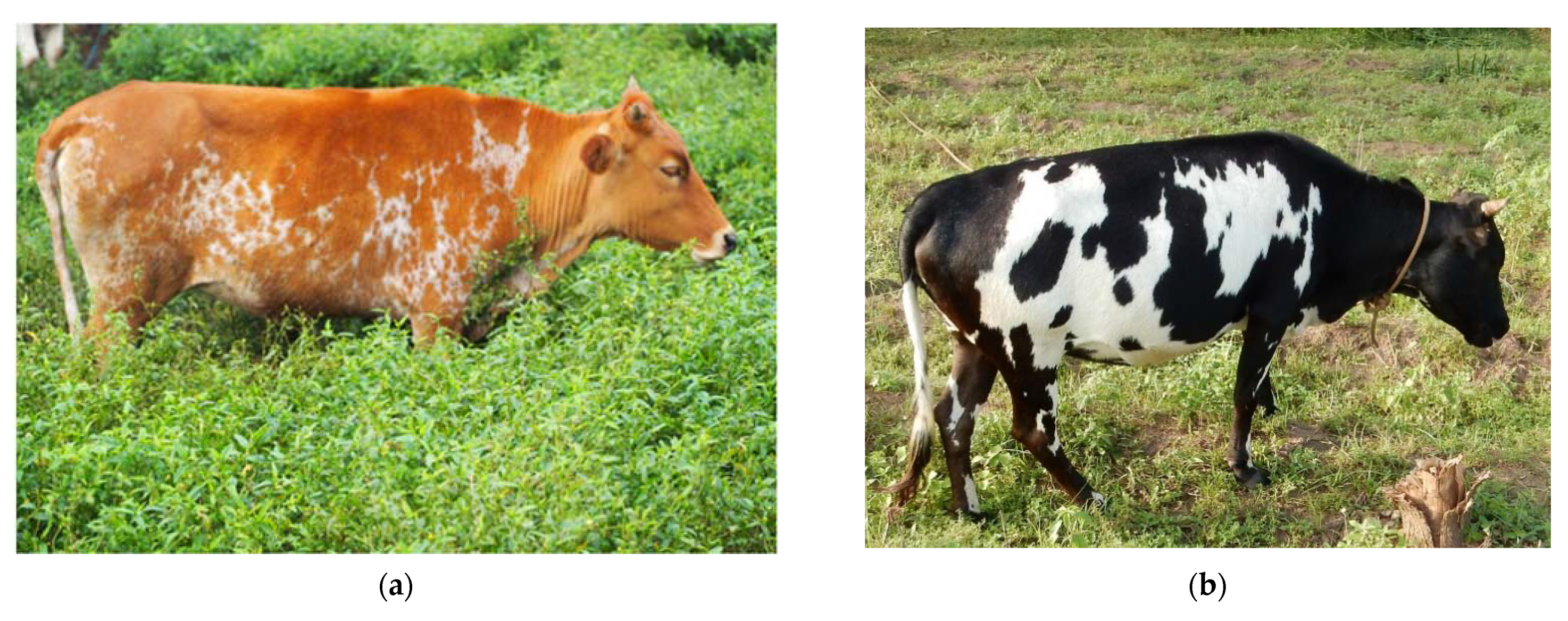This is a detailed description based on three different captions of two photographs placed side by side, showcasing two distinct cows, labeled A on the left and B on the right. 

In Photo A, there is a brown cow with white spots, standing in an overgrown meadow with grass up to its knees. The cow is facing right in a profile view, revealing wrinkled skin around its neck and jaw. Noteworthy is a small horn covered in fur on the top of its head. The cow's rust-colored body features white splotches primarily along its belly, rear hip bones, and extending up its back.

Photo B features a smaller, jet-black cow adorned with white patches, particularly noticeable under its belly, on its right shoulder, and near the back legs. The cow also has a white patch on the rear part of its tail, with a section of long black hairs at the tip. A thin rope, resembling a leash or collar, is tied around its neck. This cow also faces right in a profile view and is grazing on short grass in a less dense, green field. Both cows are situated in lush, green environments, though the grass in Photo A is much taller than in Photo B.